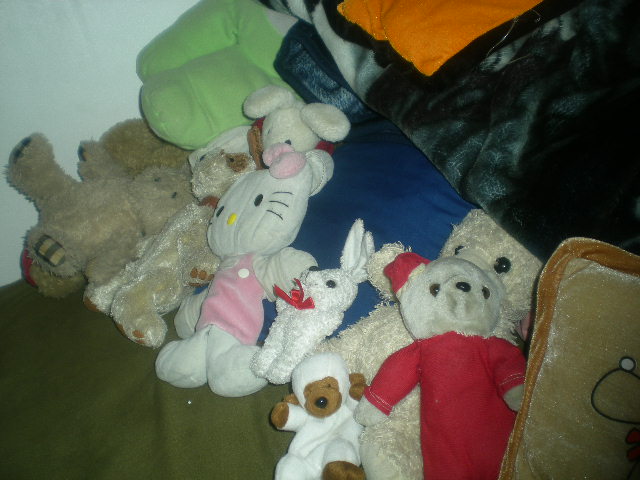The image displays a cozy bed adorned with a diverse collection of approximately a dozen stuffed animals. The setting is a child's bedroom, providing a plush and inviting background. The bedding features a dark green blanket and a light blue pillowcase, complemented by an orange blanket with a black outline. Prominently, there's Hello Kitty in a pink dress with a pink bow, a white bunny with a red ribbon and black beady eyes, and a cream-colored teddy bear donning a red dress and a red hat. Among the assortment, there's also a white and brown dog, a gray bunny with a bumblebee-like pattern on its feet, a sheepdog with white fur and brown paws, and another red teddy bear perched on top of the first one. Each stuffed animal exhibits black beady eyes, adding to their charming appearance. The photograph exudes warmth and comfort, portraying a welcoming space for a child to enjoy.